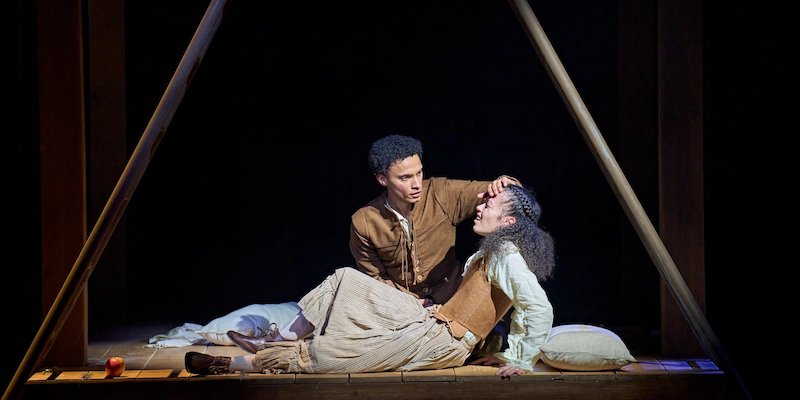In this detailed scene captured from a stage play, we observe two characters dressed in period-appropriate attire under focused artificial lighting that dramatically contrasts with the black background. The central figures are an African-American man and a woman, both with thick curly black hair. The woman's hair features a braid crowned around her head. She is reclined with a distressed expression, propped up by a pillow, and wears a long-sleeved cream-colored shirt, a leather vest, and a ruffled tan skirt with leather booties. The man, dressed in a deerskin-like brown leather jacket, sits behind her, tenderly placing his hand on her forehead as if checking for a fever. Her white shirt and brown cincher accentuate her peasant-like appearance. Just in front of her feet, an apple adds a curious element to the scene, and they are both within the confines of a wooden triangle. The compelling use of light and shadow enhances the emotional gravity of their performance.